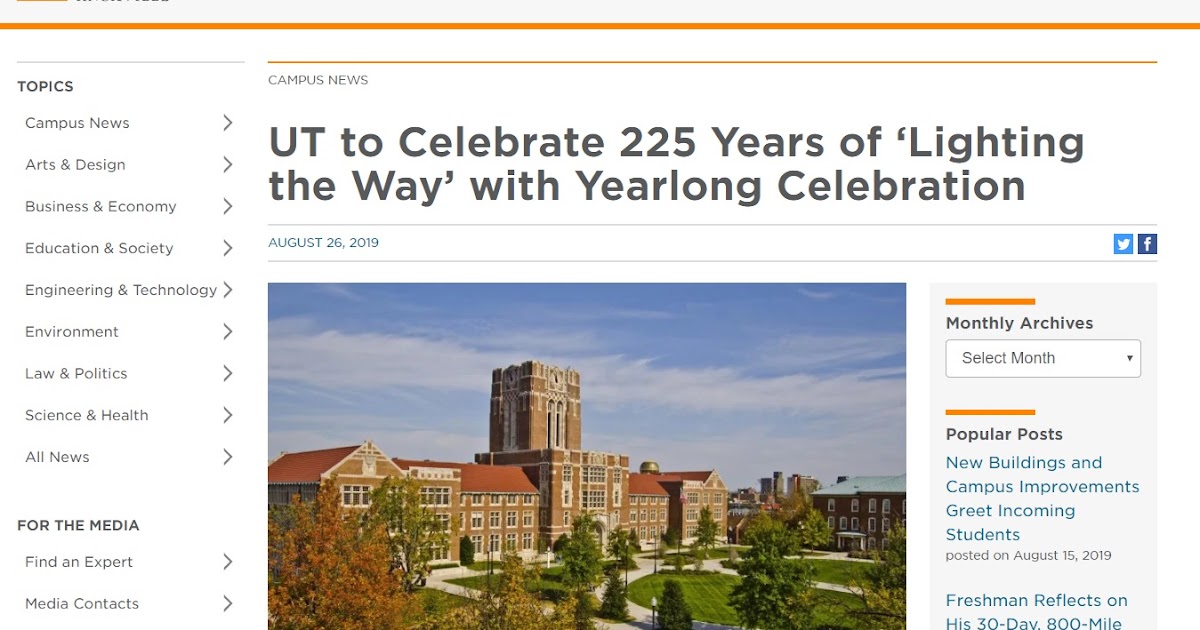The image is a comprehensive screenshot of a newspaper website, likely belonging to the University of Texas Campus News. At the top center of the webpage, the title of the featured article is prominently displayed: "UT to celebrate 225 years of lighting the way with year-long celebration." This article was published on August 22, 2019. Below the headline, there is a clear photograph showcasing the main administrative building and courtyard of the University of Texas, symbolizing the core of the university's heritage.

On the left-hand side of the page, there's a vertical navigation menu. The top section of this menu is labeled "Topics." Under this heading, there are nine clickable subtopics, each accompanied by a right-pointing arrow: Campus News (the current section), Art and Design, Business and Economy, Education and Society, Engineering and Technology, Environment, Laws and Politics, Science and Health, and All News. Just below this, another section titled "For the Media" features two subtopics: Find an Expert and Media Contacts.

The right-hand side of the page is dedicated to the "Monthly Archives" section, with a rectangular box labeled "Select Month" featuring a drop-down arrow for easy navigation through past articles. Directly below this section, there is a "Popular Posts" list, highlighting recent and noteworthy articles in blue text. The first post is titled "New Buildings and Campus Improvements Greet Incoming Students," published on August 15, 2019. The second listed title begins with "Freshman Reflects on His 30-Day 800-Mile," but the remainder of the title is cut off.

An orange horizontal line spans the top of the webpage, adding a touch of the university's school colors to the layout. The screenshot does not include any additional text beyond this detailed description.